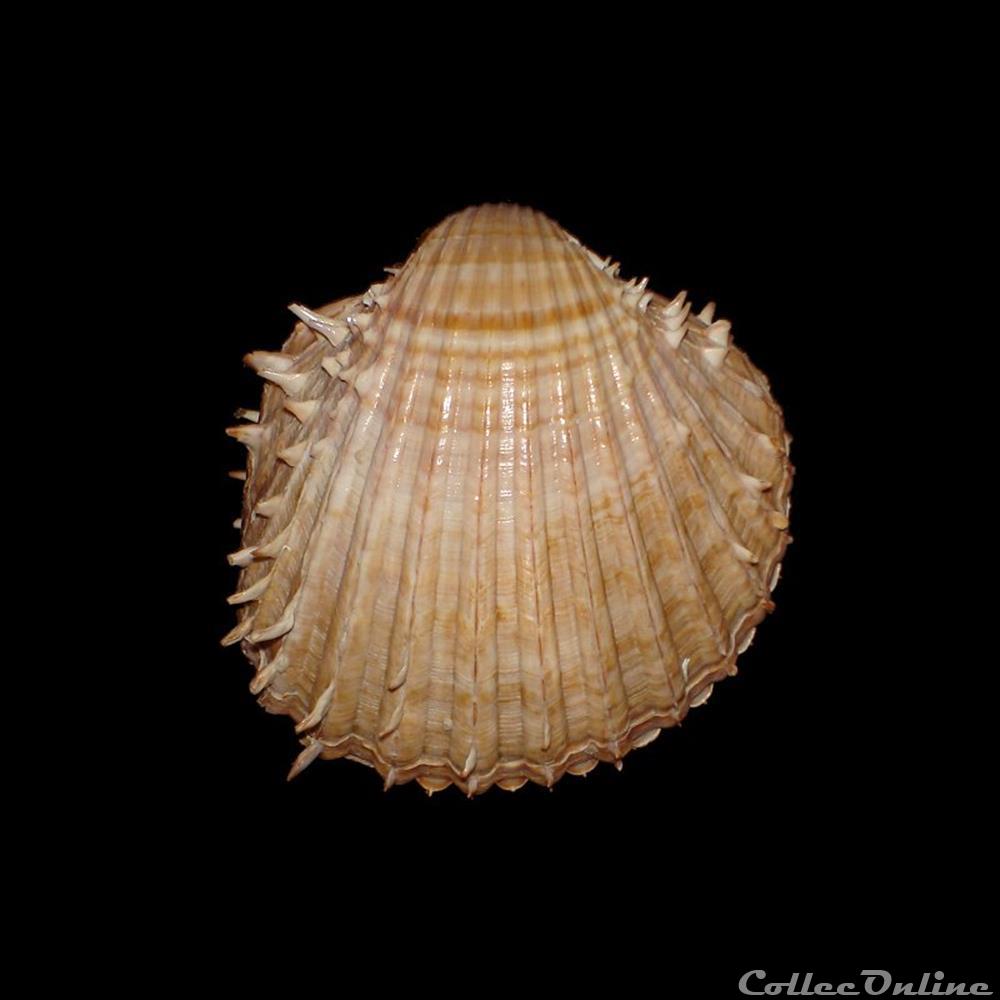This detailed color photograph captures the close-up of a seashell, possibly that of a scallop, set against a solid, very black background. The seashell, positioned perfectly in the center of the image, boasts an alternating pattern of brown, light brown, dark brown, cream, and white stripes, creating a subtle gradation of hues. The shell itself is oval-shaped, tapering to a slight point at the top, and features a series of ridges extending from its central hinge down to its broader base. Distinctively, the shell has small, pointed spikes emerging from its left and right sides, with a few more protrusions at the bottom, enhancing its textural complexity. The edges are scalloped and slightly pointed, adding to the intricate detail of the image. In the bottom right corner, out of the main focus, gray text reads "Collee online" or "Collie online," though the exact spelling is unclear due to the stylization. This shell, with its earthy tones and rich textures, suggests a moment captured by someone who may be a beachcomber, a seashell collector, or a marine biology enthusiast.